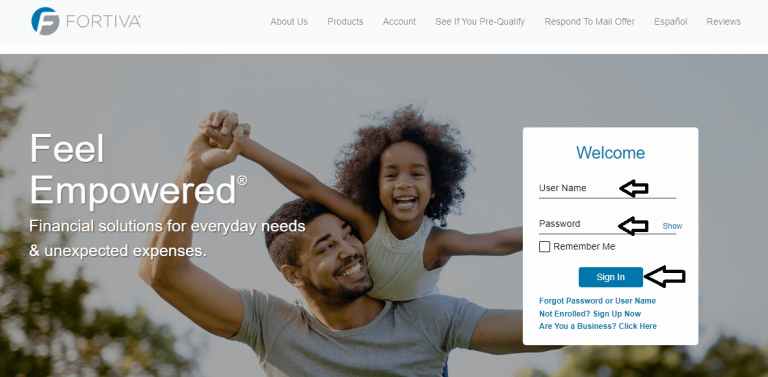The image depicts a login screen for "Feel Empowered," a financial solutions website offering services for everyday needs and unexpected expenses. The top left corner features a mix of blue, gray, and black colors. The screen prompts users to see if they pre-qualify, with an option to respond to a mail offer, including Español reviews. 

In the forefront, a person with short, slightly curly hair is holding a gray shirt, with an empowering and confident demeanor. To the right, a white window displays a username and password entry form with blue text welcoming the user. Arrows point to the username, password fields, a "Remember Me" checkbox, and a "Sign In" rectangle button. Additional options include "Forgot Password or Username,” “Non-enroll,” and “Sign Up Now.” There is also a link for businesses to click for more information.

Overall, the image conveys a message of empowerment, emphasizing user-friendly financial solutions and account accessibility.